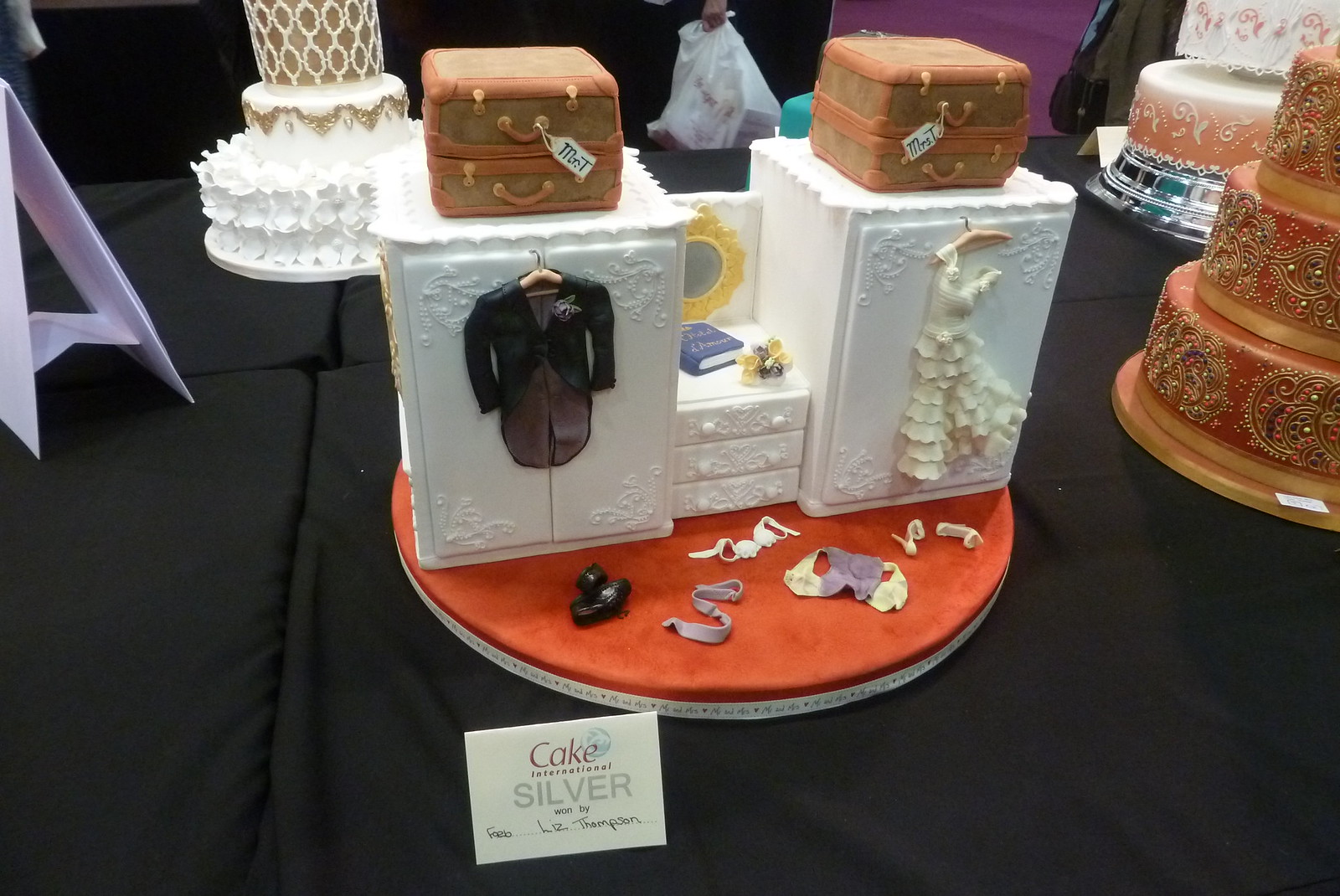This intricate photo captures a detailed cake that is crafted to resemble a wedding scene. The main feature is a wardrobe-themed cake centerpiece set atop a circular red cake stand or tray. On the left of this central cake is a tall wardrobe with a sleek tuxedo jacket hanging inside, and a suitcase labeled "Mr. T" placed on top. To the right, there is an elegant, frilly wedding dress hanging from another wardrobe, also topped with a suitcase labeled "Mrs. T." In the center between these wardrobes is a three-drawer dresser adorned with a mirror, a small purple book, and some flowers on top. Scattered around the base of the wardrobes are various discarded garments, including shoes, a tie, a bra, and a vest, suggesting the aftermath of a wedding celebration. This ensemble rests on a black tablecloth, surrounded by other ornately decorated cakes, showcasing the delicate craftsmanship and intricate patterns. A name tag in front of the main piece indicates it might be part of a display, possibly in a bakery or a cake decorating competition.